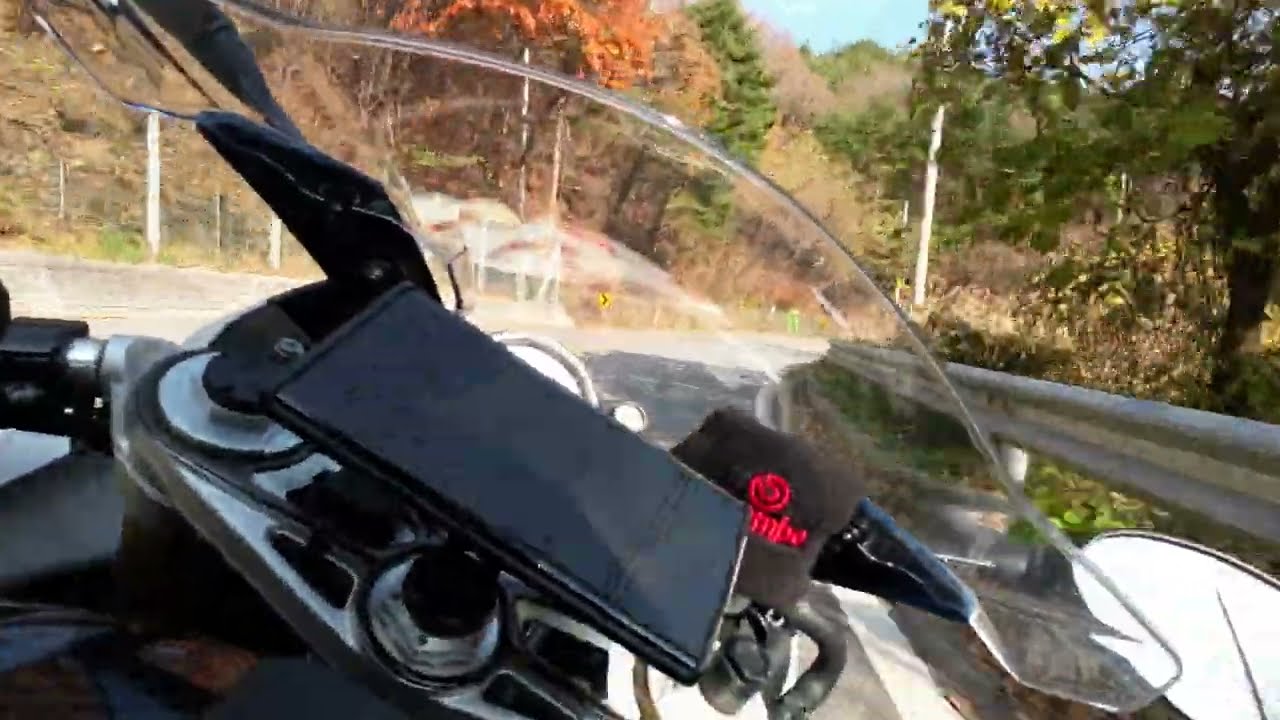The point-of-view image captures a motorcyclist's perspective while leaning slightly to the right on a curved, light gray road with white markings and silver metallic railings on both sides. The center of the image is dominated by the motorcycle's handlebars and a small, curved, clear windshield. A smartphone is mounted on the center console next to a black wristband with red writing and a red circle. Surrounding the road is various vegetation, including trees with leaves in vibrant shades of orange, yellow, green, and tan, indicating a fall setting. The sky overhead is a clear, light blue with no clouds in sight. Additionally, mirrors are visible on either side of the motorcycle's handlebars, contributing to the detailed capture of this scenic autumn ride.